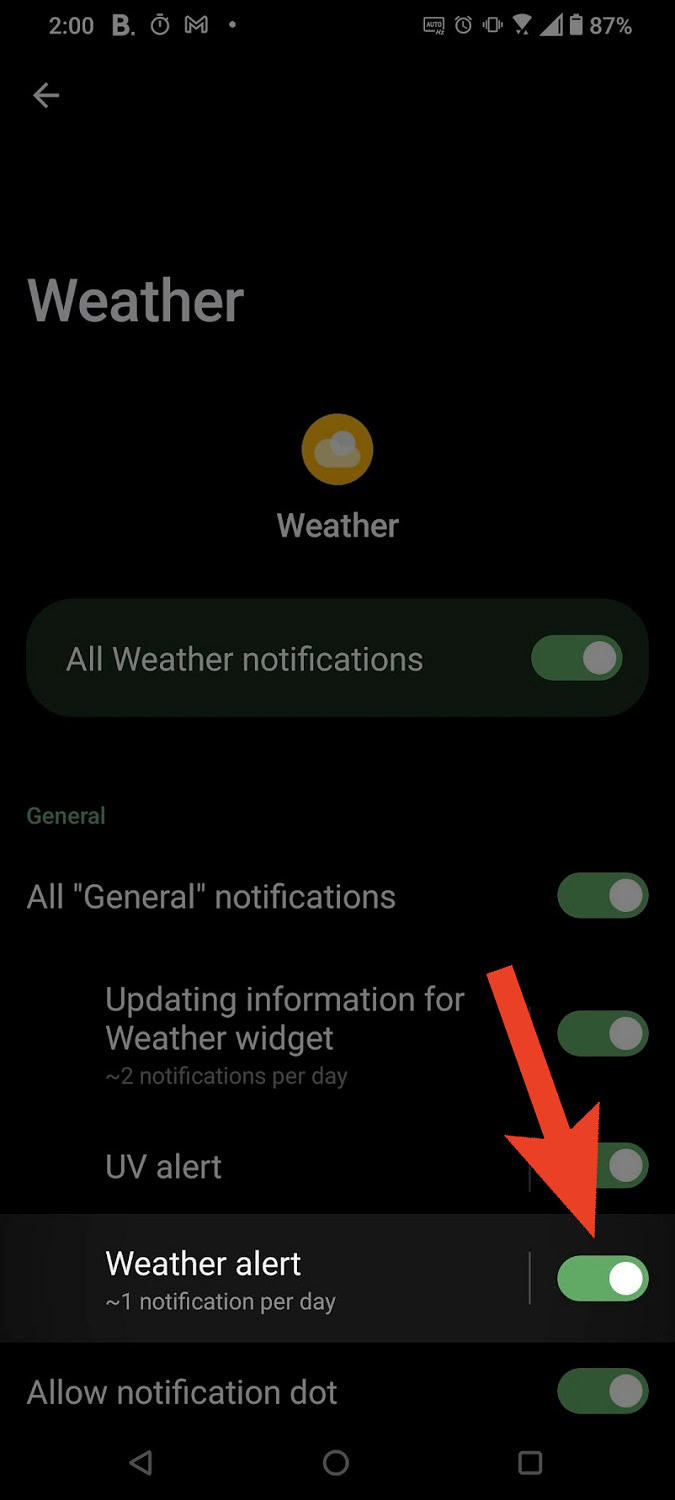This image is a screenshot taken from a mobile phone, identifiable by its elongated, rectangular dimensions and the typical status icons at the top. The top bar displays a multitude of icons: a clock showing 2:00, an alarm clock symbol with a letter 'B' next to it, the Gmail icon, another alarm clock symbol labeled ‘AUTO,’ Wi-Fi signal strength, and a battery icon indicating 87% charge.

The central part of the image appears to be a tutorial or configuration guide for a notification system. It features a series of options under categories titled "Weather" and "General." Each category contains toggle switches. The "All Weather Notifications" option is toggled on, as indicated by the green switch with a white slider. Similarly, "All General Notifications" is also enabled, with the same green-and-white toggle button.

Highlighted in this image is a specific notification setting: "Weather Alert." This option specifies that one notification per day is activated, providing a detailed level of customization for the user. All the text within the image, apart from the highlighted green toggle switches, is white, contributing to a clear and readable interface.